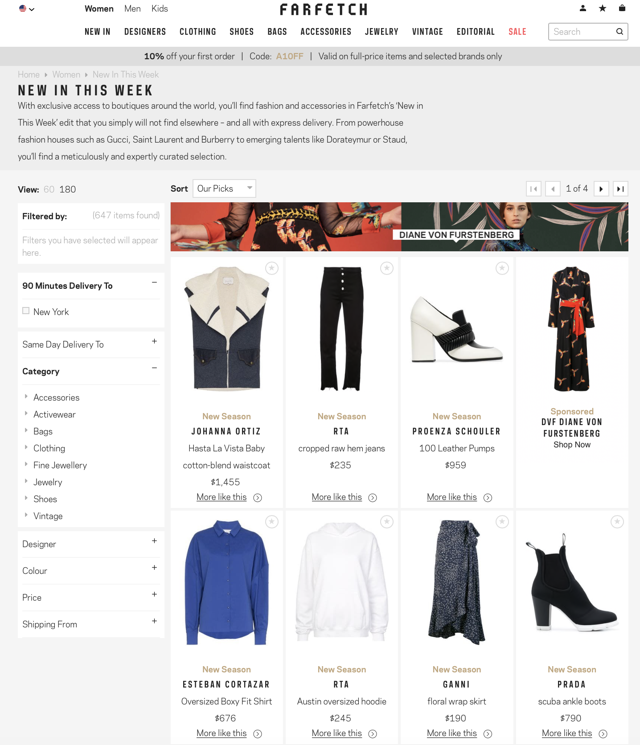This is an image of the Farfetch website, showcasing its layout and offerings. At the top-center of the image, the Farfetch logo is prominently displayed. To the left of the logo, the navigation menu begins with the word "Women" in bold black letters, highlighted to indicate the current selection. Adjacent to it, "Men" is written in bold gray letters, followed by "Kids" in the same bold gray font towards the right. 

Below this primary navigation, additional headings are listed in bold black letters: "New In," "Designers," "Clothing," "Shoes," "Bags," "Accessories," "Jewelry," "Vintage," and "Editorial," each representing a clickable category. The word "Sale" stands out in bold red text, offering an emphasis on discount items. To the far right of these headings is a search bar for user convenience.

Directly underneath this navigation, a promotional banner reads "10% off your first order. Code A10FF," with a note to the right that specifies the offer is "valid on full price items and selected brands only."

Further down the page on the left side, "New in This Week" is displayed in bold black letters, introducing a curated selection of the latest fashion pieces. The accompanying text explains that Farfetch provides exclusive access to boutiques worldwide, offering unique items that are delivered with express service. It highlights luxury brands like Gucci, Saint Laurent, and Burberry, as well as emerging designers such as Dora Tamer and Stowed.

Below this introduction, a "View" filter appears in bold black letters, next to which are the light gray number "60" and darker gray number "180." "Filtered by" is then listed in bold black letters, followed by "646 items found" in gray lettering, which indicates the number of available items. Below this, an advisory note states that "filters you have selected will appear here."

Moving further down, the section highlights service specifics like "90 Minutes Delivery" in bold black letters with an unchecked box next to "New York," indicating this service is available in the city. Similarly, "Same Day Delivery" is noted in black letters, accompanied by a plus sign to expand further options.

In the leftmost column, "Category" is displayed in bold black letters with a minus sign for collapsing or expanding the list. Subcategories include "Accessories," "Activewear," "Bags," "Clothing," "Fine Jewelry," "Jewelry," "Shoes," and "Vintage," each listed in gray text.

Further categorization options include "Designer," "Colour," "Price," and "Shipping From," each highlighted in gray text with a plus sign for additional filtering.

To the right of these filtering options, a box displays thumbnail images of eight products, presumably showcasing some items from the curated selections or new arrivals.